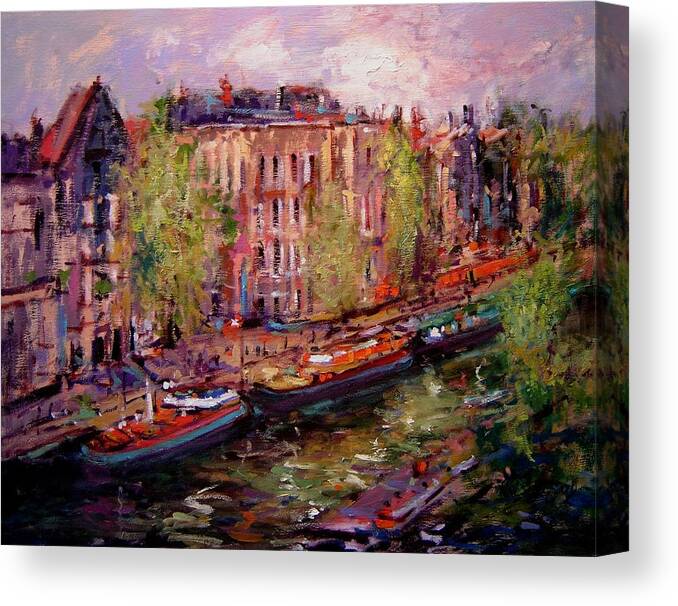This captivating impressionistic oil painting, reminiscent of Monet's style, depicts a European canal city, likely in the Netherlands or Italy. The landscape is richly adorned with vibrant colors, particularly pink, purple, and green, which lend a dreamy quality to the scene. The cityscape features towering pinkish-brown buildings with red roofs, complemented by lush green trees in the foreground and background. The canal itself is framed by both a walkway and verdant greenery on either side, contributing to the serene ambiance.

The dark waters of the canal are populated by about six boats in vivid hues: a red boat, a yellow boat, a green boat on the left, along with a reddish and a bluish boat on the right. Small, delicate figures can be seen standing along the canal, adding a sense of scale and life to the painting. The sky, awash with purples and accented by white clouds, suggests a twilight or early evening setting, enhancing the painting's tranquil and somewhat romantic atmosphere. The artwork is executed on canvas, with a distinct perspective that makes the scene appear to recede gently to the right, giving it a slightly three-dimensional effect. This piece captures the essence of a serene canal city, celebrating both architectural and natural beauty through a harmonious blend of colors and impressionistic technique.